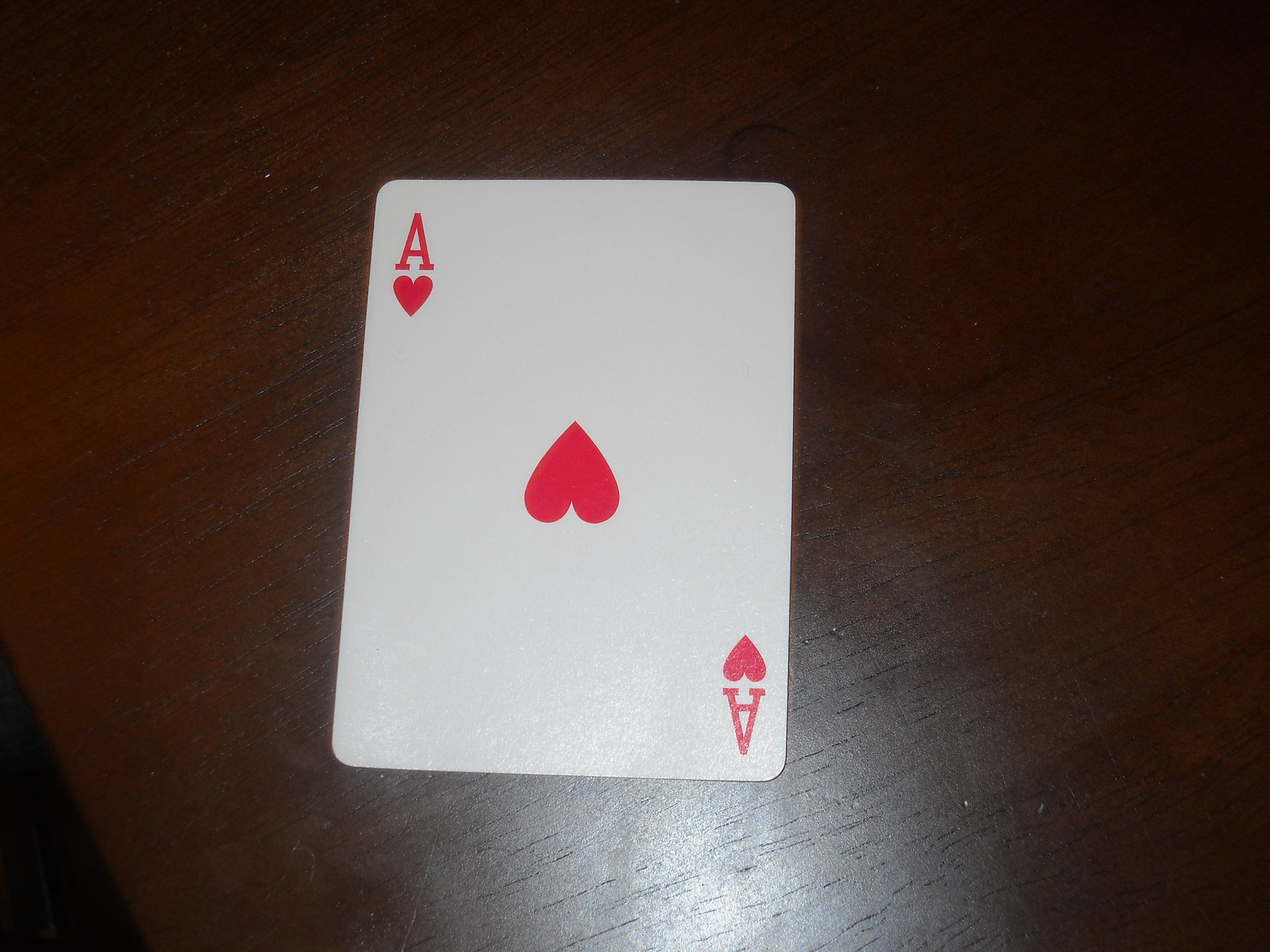In the image, a single playing card, the Ace of Hearts, is prominently displayed on a dark wooden table. The photograph is a close-up shot taken from above, capturing the fine details of the card and the rich texture of the table. The Ace of Hearts is positioned such that its value and suit symbols—a red 'A' and a small heart—are visible in the top left and bottom right corners of the card. In the center of the card, an upside-down red heart further indicates that the card itself is oriented upside down. The bottom right corner of the image reveals the edge of the table, dropping off into a deep black void, adding a dramatic contrast to the scene. The card's slightly rectangular shape and traditional design are clearly visible, making this a classic representation of a playing card in a striking setting.